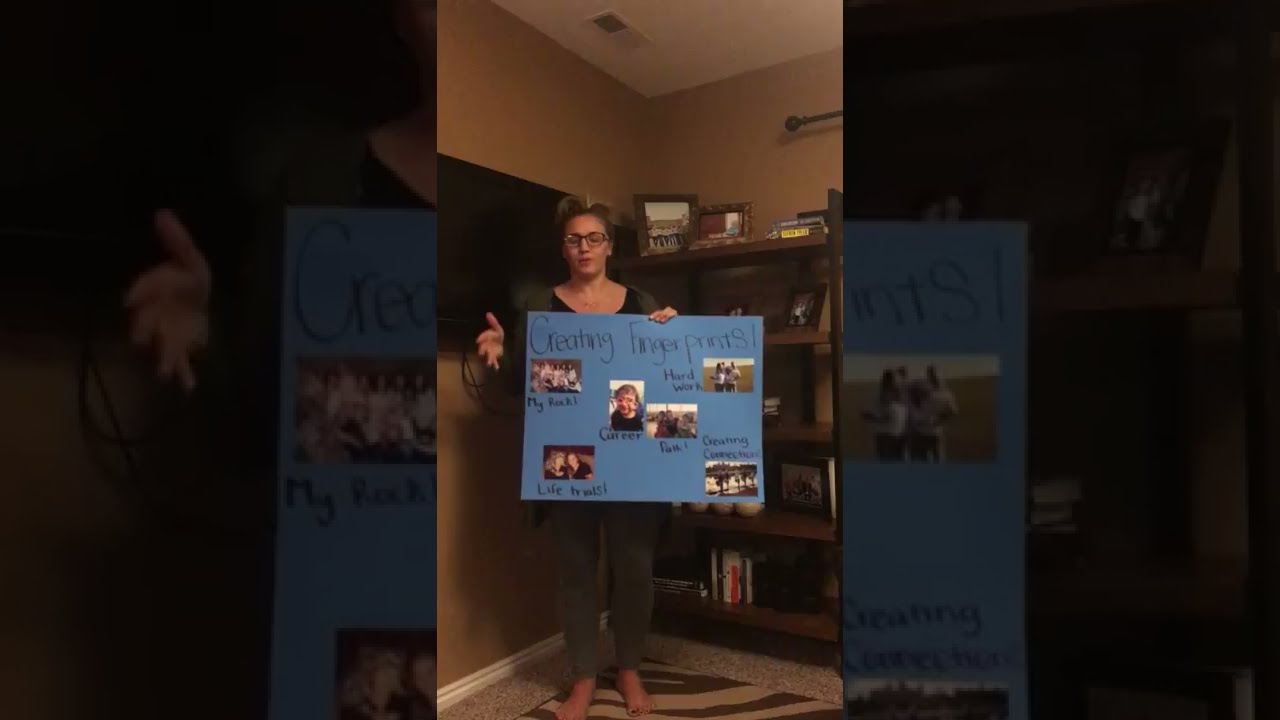In the photograph, a middle-aged woman with light brown hair and glasses stands in front of a bookcase, holding up a handmade blue crepe paper poster. She is wearing a black shirt under a green sweater. The poster, titled "Creating Fingerprints," features six photographs each with a caption underneath them, though some of the captions are difficult to read. The upper left photo reads "My Something," followed by "Career," "Path," and "Hard Work" on the top row. On the bottom row, it reads "Life Trials" and "Creating Corrections." Each photo depicts different aspects of life, including groups of women, an individual, a family in a field, two smiling women, and a lake surrounded by trees. The image also features black bars on either side of the person, which make up about two-thirds of the total image. To the left of the woman, there appears to be a computer screen or a small TV mounted on the wall.